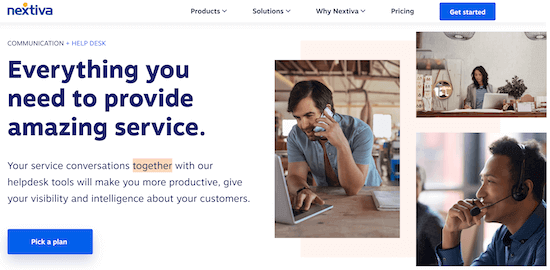The website features the logo "Nextiva" in blue located in the top left corner, with an orange circle positioned above the "X" in the logo. Adjacent to the logo, there is white space followed by a series of navigational links: "Products" with a downward arrow, "Solutions" with a downward arrow, "Why Nextiva" with a downward arrow, and "Pricing." On the far right, there is a "Get Started" button displayed in white font against a blue rectangle.

Below this navigation bar, three images are displayed. The first image shows a man holding a phone to his ear. He is dressed in a blue button-up shirt and a beige tie. He has black hair, neatly parted and swept to one side. He appears focused, with one hand on a laptop keyboard as he looks at the screen.

The second image features a woman sitting at a desk with a laptop in front of her. She is examining some papers spread out on the table. A circular mirror is mounted next to her on a shelf, and lights are visible overhead, illuminating her workspace.

The third image depicts a man wearing a headset with a microphone near his mouth. He has short, curly hair, and darker skin, and he is dressed in a blue long-sleeve button-up shirt. His hand rests thoughtfully against his lips.